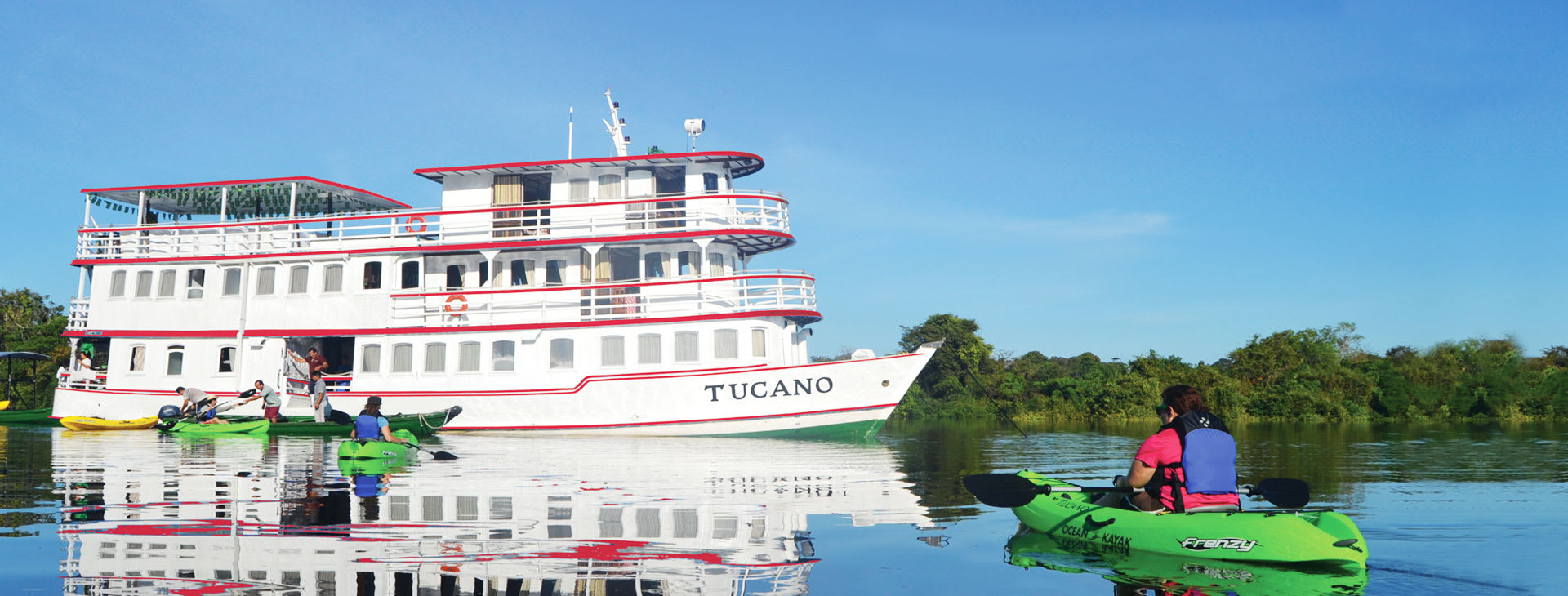This vibrant and symmetrical photograph captures a scene on a serene river with a striking bright blue sky overhead. The centerpiece is the large, three-deck tour boat named "Tucano," featuring a predominantly white hull with vivid red lining and railings on each level, topped with equipment near the captain's room. In the foreground, the water mirrors the sky's robin's egg blue hue and the deep green foliage lining the riverbanks. Around the boat, several brightly colored kayaks populate the river—mostly light green and yellow—with each kayaker donning a blue life jacket. Notable among them is one kayaker on the left, identified with a "Frenzy" kayak. The kayakers, who may have embarked from the tour boat for recreation, add to the lively, multicolored aspect of the scene. Reflections of the boat, sky, and surrounding greenery create a picturesque and dynamic waterscape.